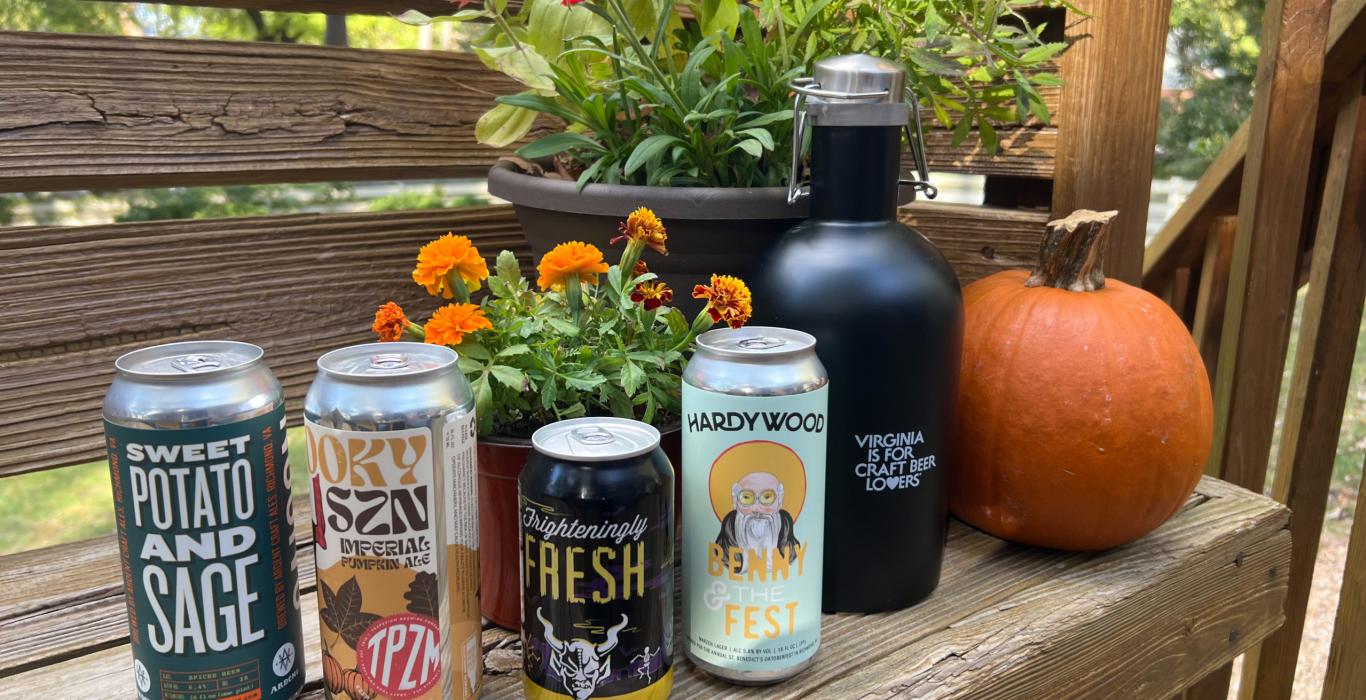The image depicts a sunny outdoor scene on a back porch, featuring a wooden bench set against a deck with wooden stairs in the background. On the bench sits a bright orange mini pumpkin, symbolizing the fall season, alongside a carafe emblazoned with "Virginia is for craft beer lovers," indicating a Virginia setting. Complementing the autumnal theme, a pot of vibrant orange mums adds a splash of color. Arranged in front of the pot are four different craft beer cans: from left to right, they include a Sweet Potato and Sage beer, an Imperial Pumpkin Ale labeled "D-O-K-Y-S-Z-N," a black can with a demonic figure labeled "Frighteningly Fresh," and a light blue can from Hardywood labeled "Benny and The Fest." The scene is bathed in natural light, with hints of greenery and tree foliage visible, reinforcing the outdoor, fall atmosphere.